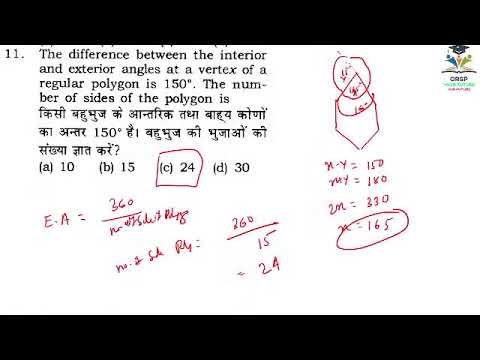The image depicts a section of an educational web page focused on a mathematical topic. The page has a black header and footer framing a white background, with the number "11" in black text in the upper left corner, indicating it is likely point 11 of a larger presentation. The main text states: "The difference between the interior and exterior angles at a vertex of a regular polygon is 150 degrees. The number of sides of the polygon is..." followed by three lines of Indian text, presumably reiterating the same question.

Below this, there are four horizontal multiple-choice options labeled A, B, C, and D. Choice C, which is the number 24, is encircled in red. Surrounding the question are red handwritten notes, indicating the person has used the page to work through the problem. The handwritten notes include equations such as "EA = 360 /" (partially obscured), "260 / 15 = 24", and others like "N - Y = 150", "N + Y = 180", "2N = 330", and "N = 165". There are also some geometrical sketches and additional symbols alongside these calculations. In the upper right-hand corner, the blurry outline of a school logo can be seen.

Overall, the image captures a detailed snapshot of a student actively engaging with a mathematical problem, complete with their problem-solving process annotated directly onto the educational web page.